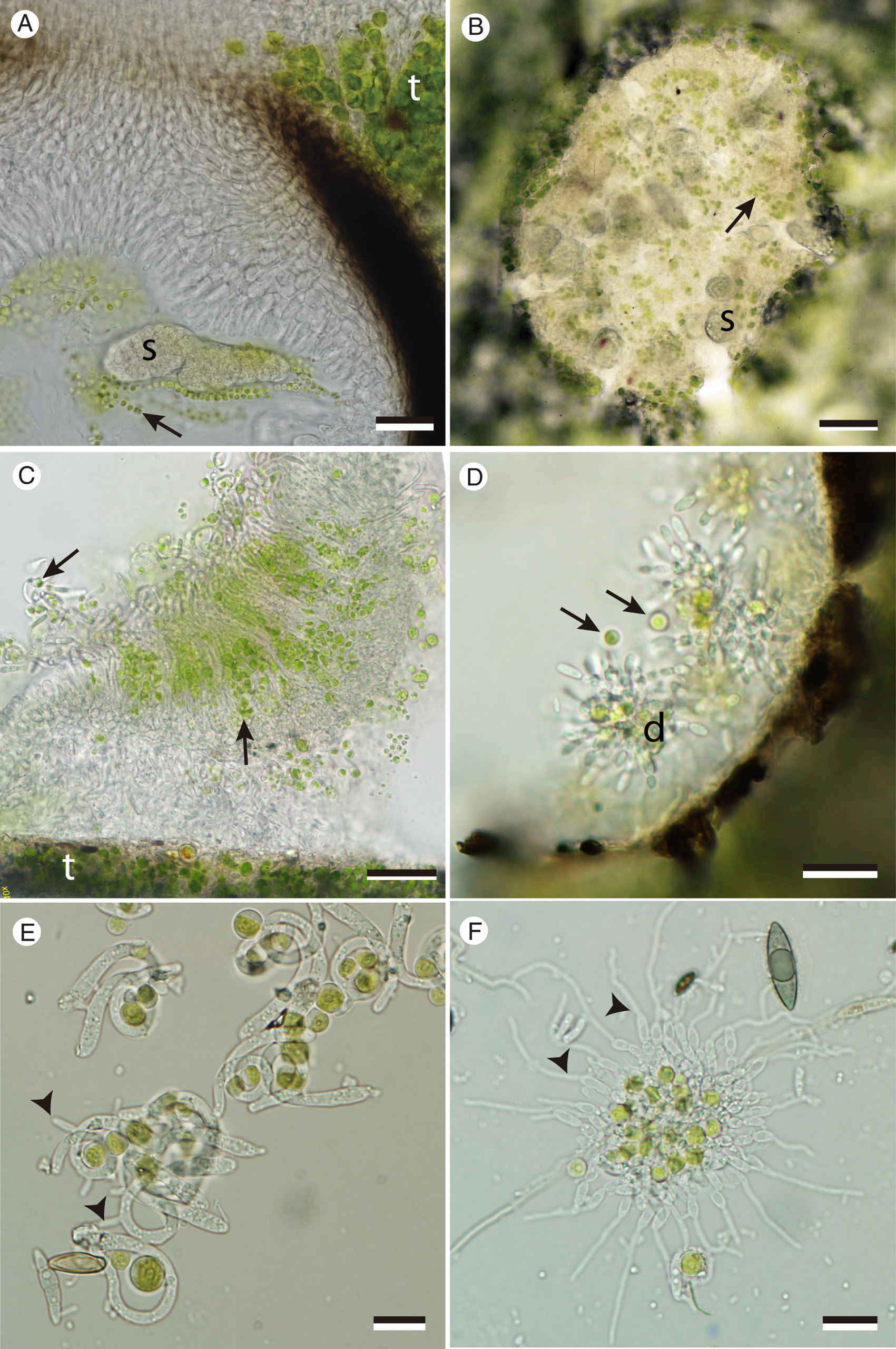The image comprises six microscopic photographs, orderly arranged in three rows and two columns. Each square image is labeled in its top left corner within a white circle, featuring a black alphabet ranging from A to F. 

The top-left image, marked with 'A,' displays a cellular structure on a grey background with a notable green area surrounding the cell, located at the bottom of the picture. Significant annotations are present, including a black 'S' atop the central cell and a white 'T' over green spores in the upper region. Adjacent to it, the 'B' image shows an elongated brown area accompanied by green, spore-like cells. 

In the middle row, the 'C' picture features a white backdrop with clusters of light green lines, while 'D' portrays white bead-like clusters against a dark green background. The third row illustrates the 'E' image on a tan background, highlighting white blobs interspersed with dark green dots. Finally, 'F' presents a grey background with light green blobs clustered at its center.

Each photograph includes arrows pointing to specific areas for detailed examination, suggesting a variety of magnifications and cellular structures under a microscope, highlighted with distinct colors and annotations.